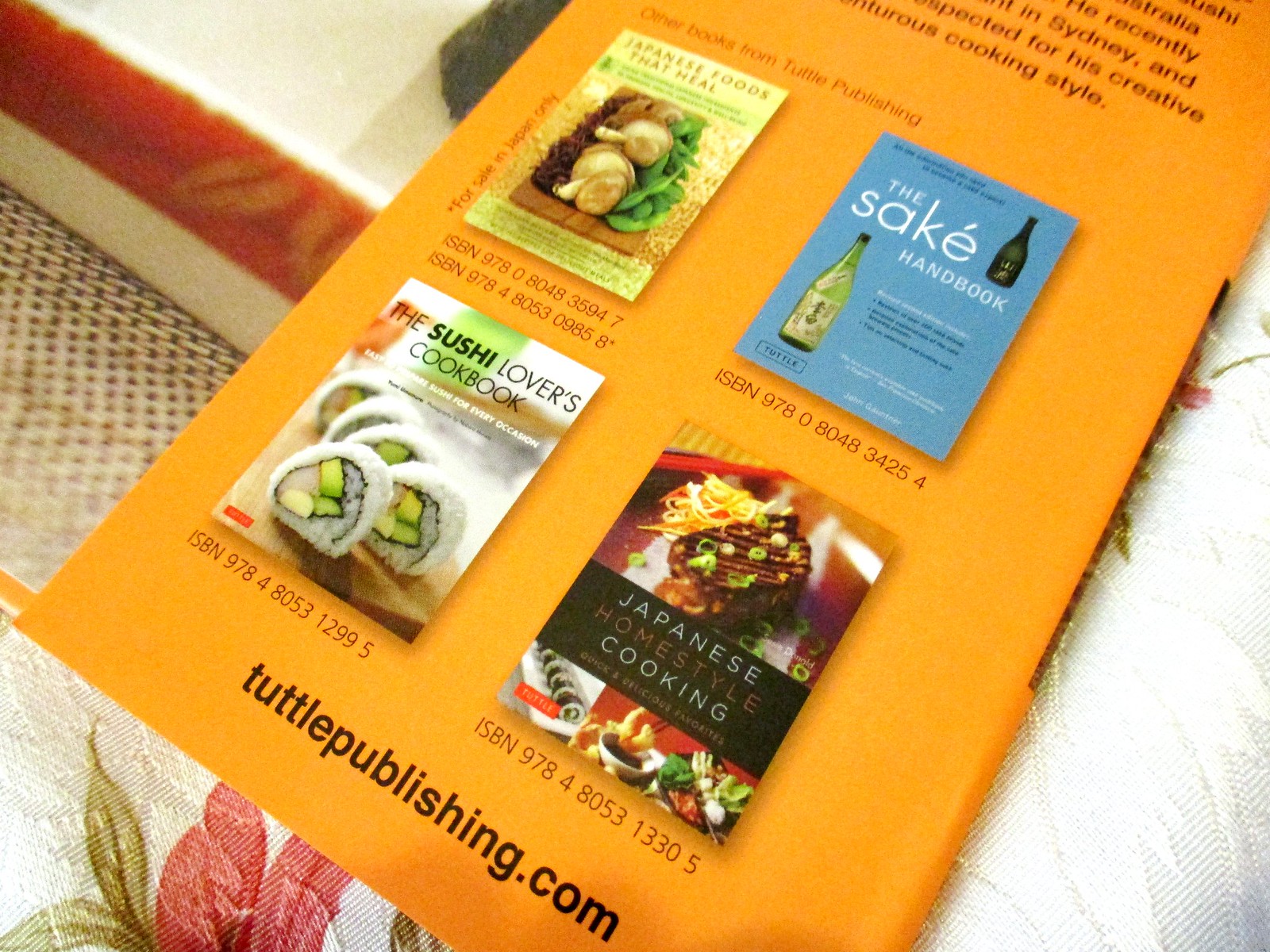This image is a detailed, color photograph showcasing an orange promotional page from Tuttle Publishing, advertising four culinary books focused on Japanese cuisine. The page is set at an angle on a cushion decorated with white, red, and green floral patterns. The page features black text at the top, followed by partially visible promotional content. The main focus is on the four book covers, arranged in two rows of two. From top left to bottom right, the books are titled: "Japanese Foods That Heal," "The Sake Handbook," "The Sushi Lover's Cookbook," and "Japanese Home Style Cooking." Each book cover includes an ISBN number. At the bottom of the page, the URL "TuttlePublishing.com" is printed in black text, indicating where these books can be purchased. The photographic style of the image emphasizes realism and attention to detail.